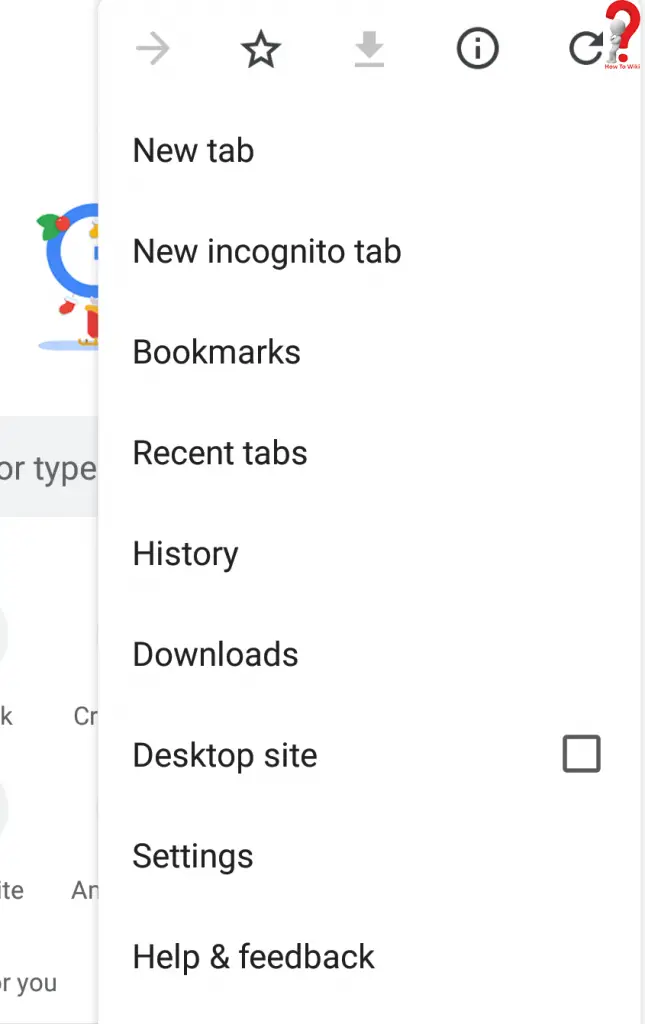The image depicts a screenshot from a mobile device showcasing a browser menu against a white background. At the top of the screen, there is a series of symbols: a light gray right-pointing arrow, a black-outlined star, another light gray arrow pointed downwards with a light gray line beneath it, a circle with a small eye inside, and a circular arrow pointing to the right. Below this icon row, there is a graphic of a little man leaning against a red question mark, accompanied by partially visible text starting with "How to W."

Further down the screen, a vertical menu lists various options: New Tab, New Incognito Tab, Bookmarks, Recent Tabs, History, Downloads, Desktop Site (with an unchecked white square to the right), Settings, Help, and Feedback. These labels and the unchecked 'Desktop Site' option indicate that the screenshot is from a mobile browser settings menu.

In the background, there is a partially visible logo featuring a blue circle adorned with red holly berries and green leaves on the left side. The circle appears to be wearing red gloves with white fur trim and is seated in a red and gold sleigh, giving it a festive, Christmas-like appearance. However, the accompanying text in the background is nonsensical and doesn't provide any useful information. There is no additional context or identifiable text apart from the described elements.